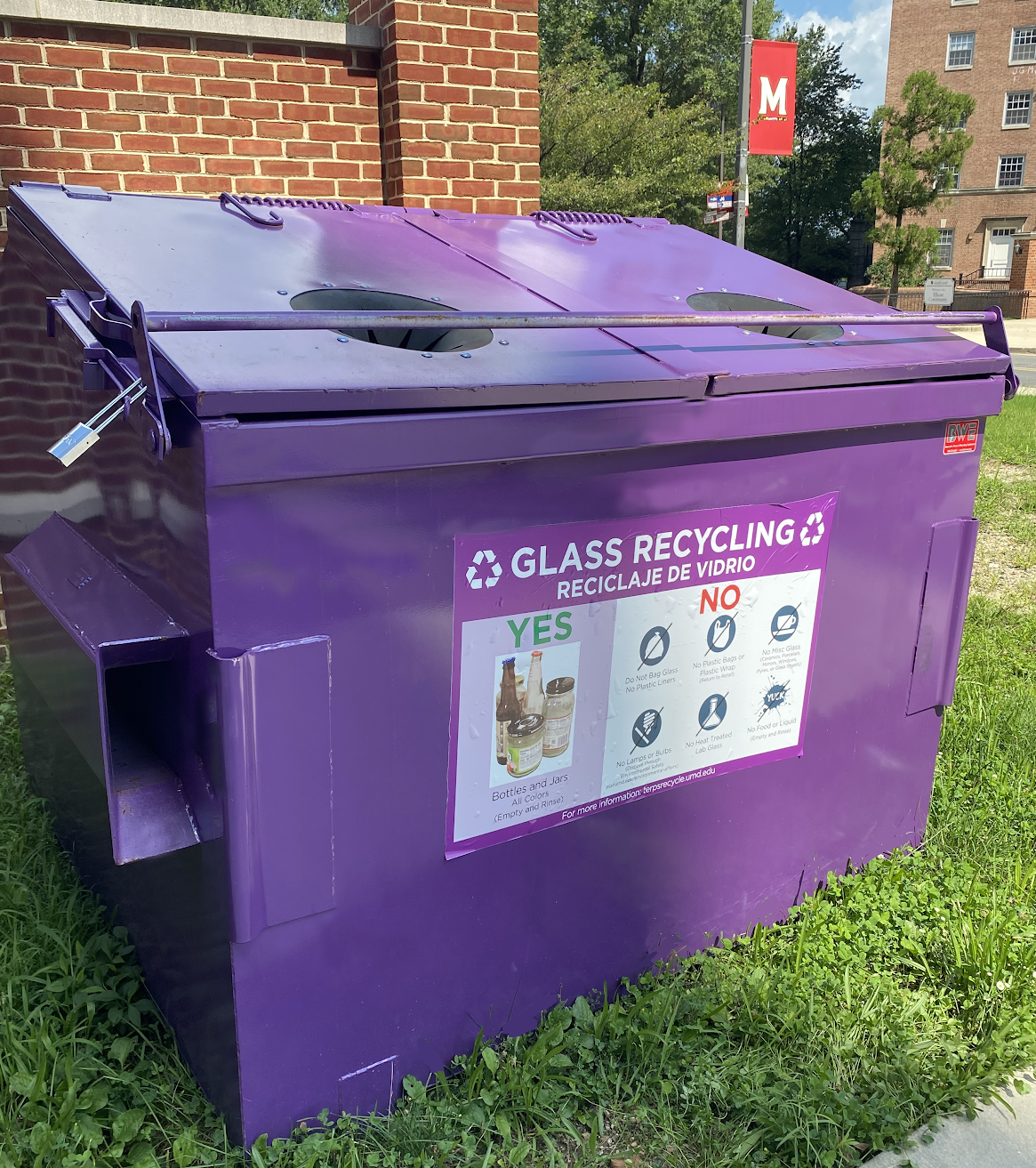In front of me is a photograph of a bright purple glass recycling dumpster. The dumpster, situated on vividly green grass, features a padlocked cover with two circular holes for glass disposal. A prominent sign on the front lists acceptable glass containers with a "yes" and items that should not be included with a "no". The side of the dumpster has a place designed for the arms of a garbage truck to lift it. The scene appears to be part of a college campus, as indicated by a banner with a large white "M" affixed to a light pole. Behind and to the side of the dumpster are brown brick buildings, one of which looks new with many windows. Tall trees can be seen further in the background. This detailed setting evokes a clean, organized area dedicated to proper recycling practices.